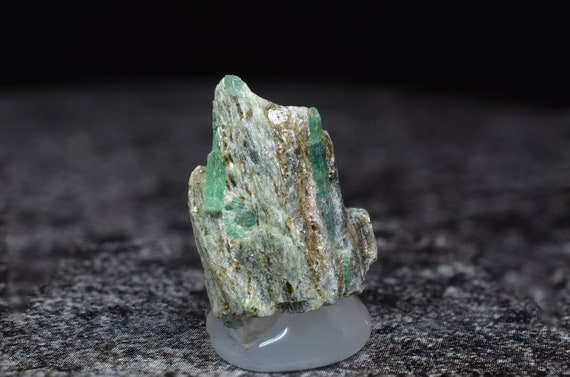The photograph captures a small, multi-colored mineral rock, prominently featuring hues of white, brown, green, and light gray, with specks of black and gold. Its shape intriguingly resembles a frog sitting upright, with a notable white circular section that looks like an eye. Atop the rock is a small green speck. The mineral is mounted on a round plastic or wax display stand, elevating it vertically. This display is set against a black and gray granite-like surface that appears in the immediate foreground, creating a stark, spotted backdrop. The rest of the surface blurs into the background, giving an impression of depth. At the top of the image is a pure black section forming a horizon with the granite. The photograph's setting suggests it might be part of a museum display or a curated collection, with the rock possibly being a special item like a gemstone or even a moon rock.